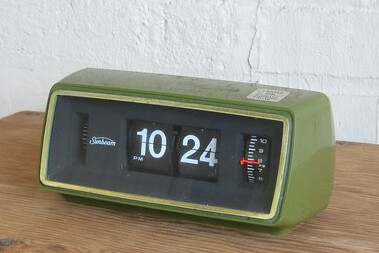This photograph captures a retro digital alarm clock, reminiscent of the 1970s, prominently positioned on a light brown wooden nightstand. The clock is set against a white wall that appears to be lined with brick or concrete. The rectangular clock has an olive green housing, with a light green outline framing its black face. At the center of the clock, white numbers display the current time, 10:24 PM, on small black plastic cards. Below the '10' is a white 'PM' indicator. The brand name "Sunbeam" is also visible on the clock face. To the right of the time display, there is an additional black dial with white numbers and hash marks, currently set to 7:45, and a small red arrow indicating the alarm time. This distinctive feature, along with the vintage design elements, underscores the clock's nostalgic charm.